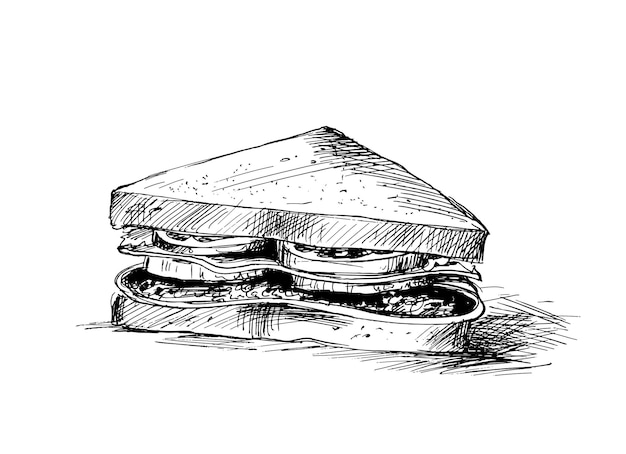This image is a black and white drawing of a triangular sandwich sitting on a scratch-marked surface that suggests a table or counter, displayed on a white background. The sandwich, seen from the side and slightly above, features detailed shading and texture indicated by black slash marks. The triangular slices of bread are clearly textured, especially along the crust. In between the two slices, you can make out layers of tomatoes, cheese, lettuce, possibly onions, and some meat, although the exact ingredients are not fully discernible. The overall simplicity of the black and white pen and ink style highlights the sandwich's structure and ingredients, making them the focal point.